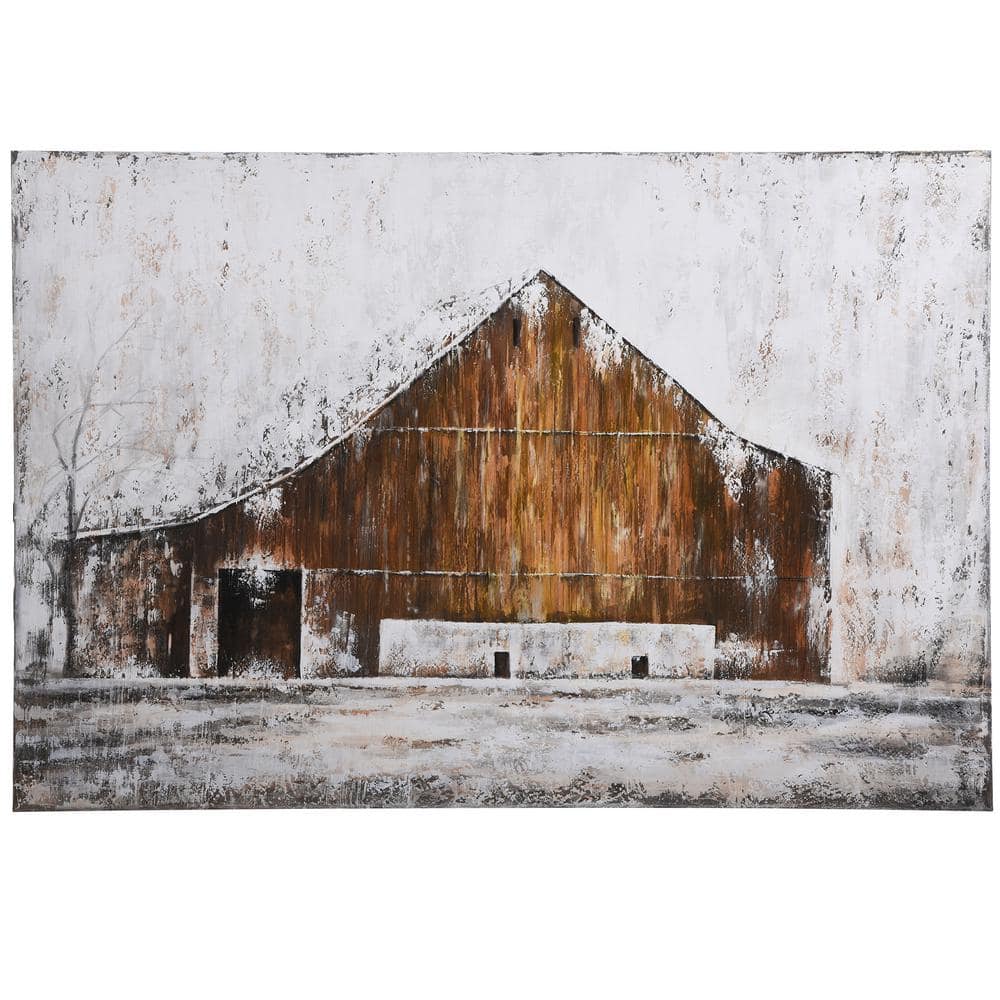A serene painting captures an old wooden barn amidst a snowy landscape, characterized by a softly textured brush technique reminiscent of gentle, brief strokes, almost as if a sponge was used. The barn, occupying a central position, is expansive with a steep, pitched roof subtly dusted with snow, indicating the wintry scene. The structure is primarily rendered in various shades of brown, from light to dark, with wooden texture discernible through the striped pattern. A distinctive feature on the barn is a white rectangle with two small black holes near the lower middle, possibly depicting a door or window. To the left, a faint, leafless tree stands, adding a touch of nature to the otherwise stark and snowy background, which spans a white, lightly snowy field merging into a whitish-gray sky, punctuated by occasional brown and gray tones. The overall ambiance suggests a quiet snowfall enveloping the rural setting.